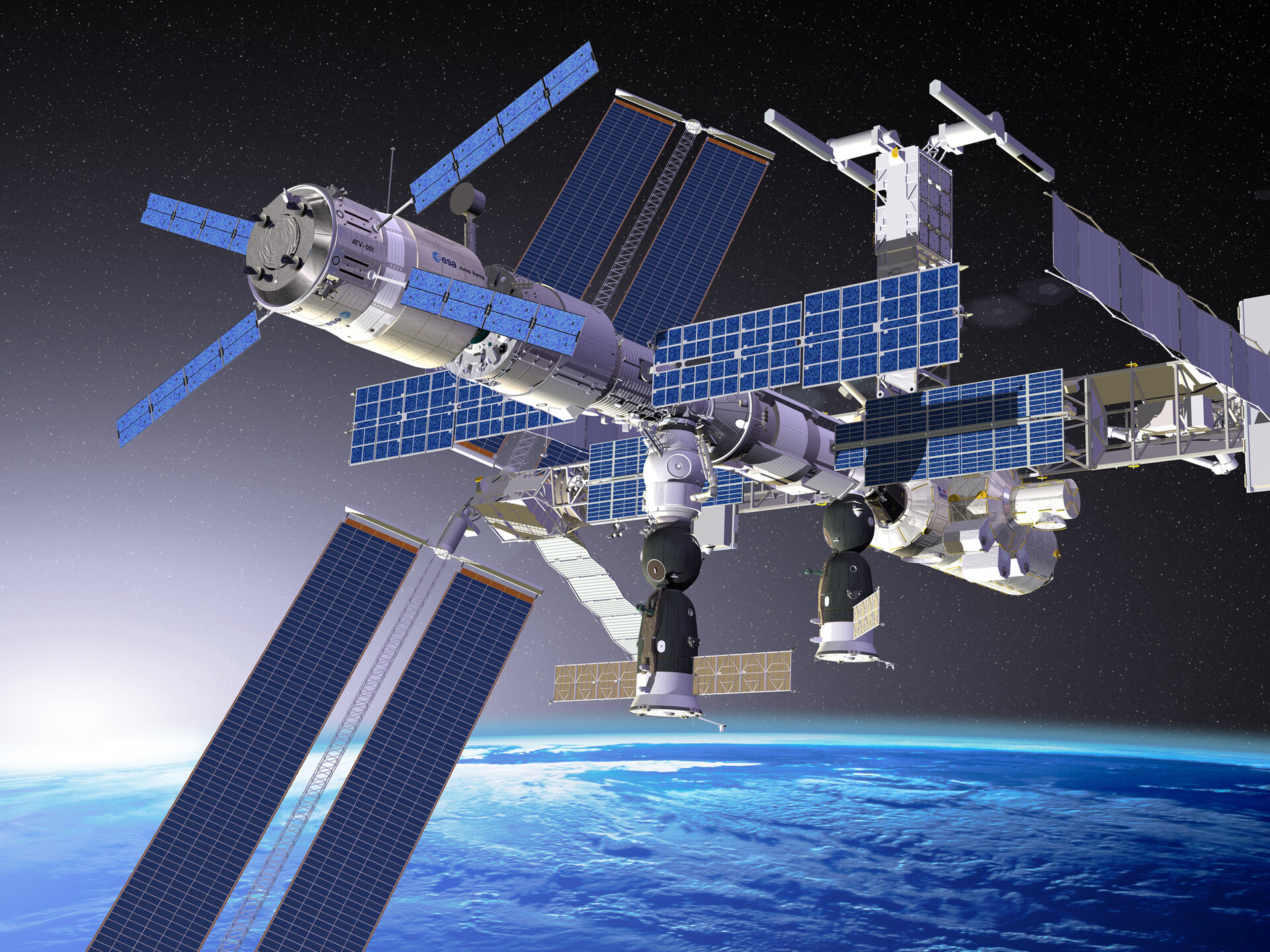The image captures a detailed, floating satellite or possibly the International Space Station, gleaming against the backdrop of outer space. The structure consists of an intricate series of cylindrical chambers colored silver and white, interconnected to form a complex network. Jutting out from these chambers are multiple grids and panels, predominantly blue and silver, which are likely solar panels. Additionally, the satellite features some dark gray and white landing feet and four small, blue rectangular grids arranged in a manner reminiscent of a static propeller. The equipment is outfitted with small cylindrical bars, possibly sonar devices, and a range of scientific instruments including docking stations and boosters. Below the satellite, Earth is visible with its vast expanses of clouds and water, while the sun peeks over the horizon on the left side, adding a brighter element to the left edge of the image. The backdrop of the scene is a deep black sky scattered with tiny white specks that represent stars, creating a vivid and awe-inspiring spatial panorama.